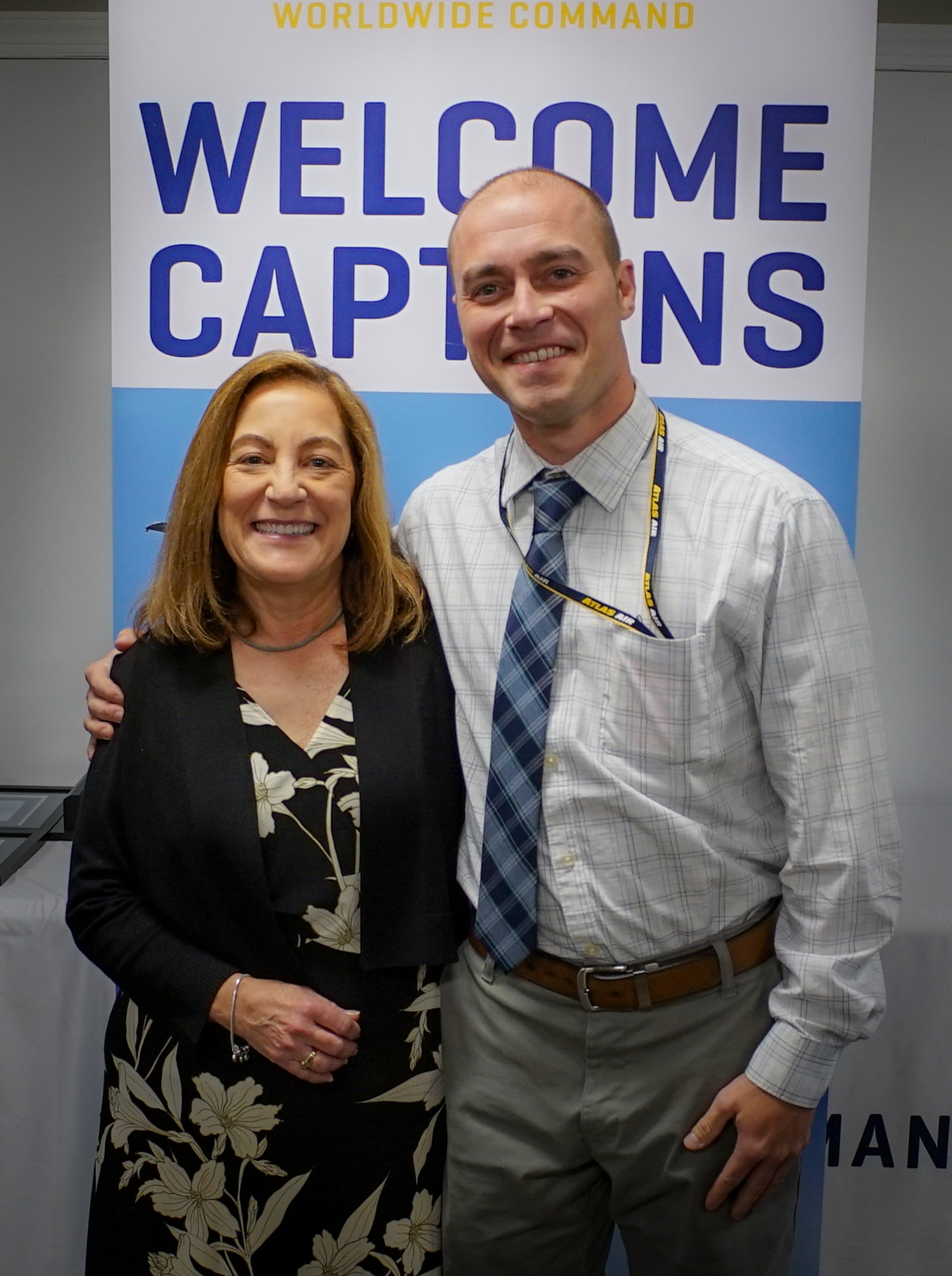The image features a man and a woman standing closely together in front of a banner. The banner, predominantly white, reads "Worldwide Command" in bold yellow letters at the top, and directly below, in large blue capital letters, it says "WELCOME CAPTAINS." Parts of the letters "T," "A," and "I" in "CAPTAINS" are slightly obscured by the man's head.

The woman, appearing older with light wrinkles, has honey blonde hair and light skin. She is smiling and wears a black cardigan over a white floral-patterned dress on a black background. Completing her outfit is a silver bracelet on her wrist.

The man, to the woman's right, has his right arm around her shoulder, conveying a gesture of camaraderie. He appears slightly younger with short-cropped hair and fair skin. He is dressed in a light-colored plaid shirt with a blue and white checkered tie. His gray slacks are held up by a brown belt, and a lanyard’s end is tucked into his breast pocket. The man has a look of around 40 years of age and is also smiling. This image suggests they might be celebrating or participating in an event related to the "WELCOME CAPTAINS" theme.